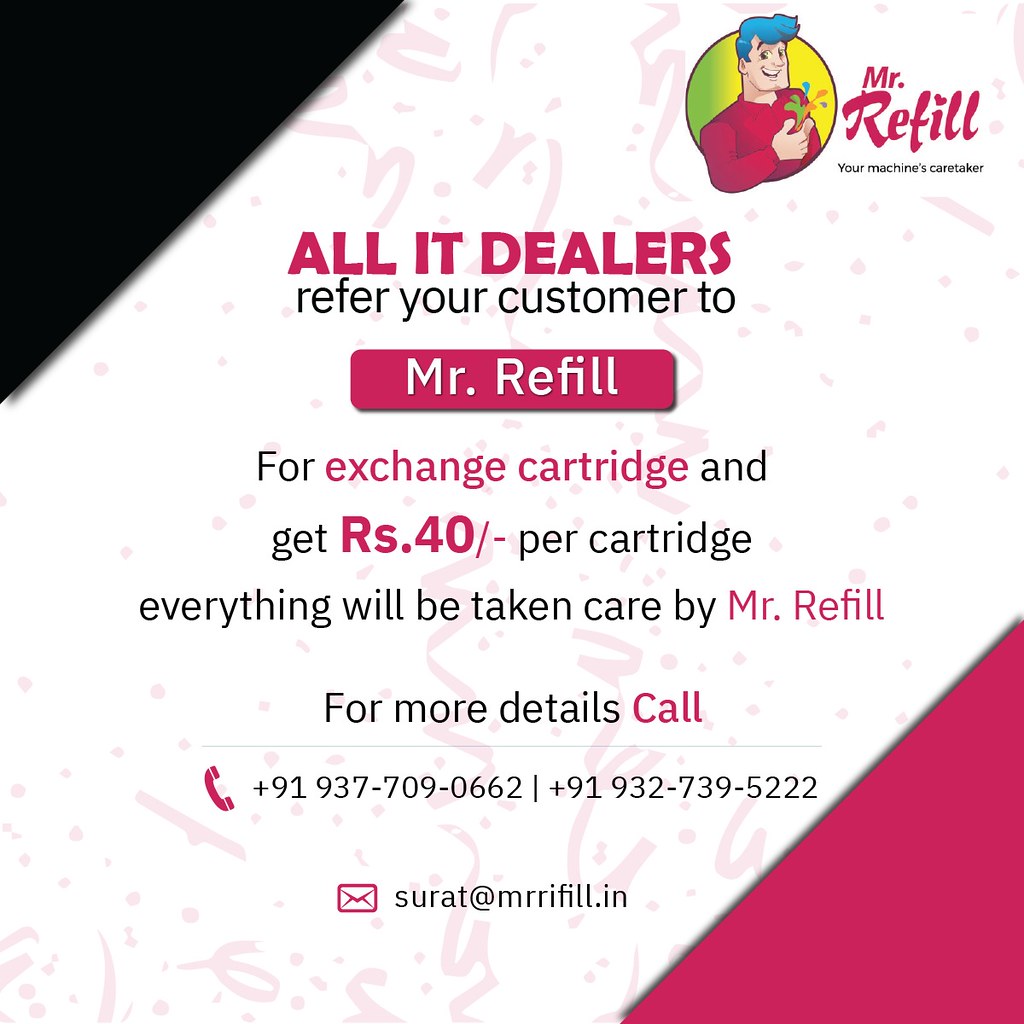The advertisement for "Mr. Refill" features a dynamic design, with a black triangle in the upper left corner and a red triangle in the lower right, framing a white center adorned with decorative red squiggles. Prominently displayed in the upper right corner is the company name, "Mr. Refill," alongside their slogan, "Your machine's caretaker," both in pink on a white background. A cartoon character with blue hair and a red shirt is also situated here, holding an object and positioned in front of a green and yellow circle.

The ad encourages all IT dealers to refer their customers to Mr. Refill for cartridge exchanges, offering a reward of RS40 per cartridge. The bold statement "All IT Dealers, refer your customers to Mr. Refill for an exchange cartridge and get RS40 per cartridge. Everything will be taken care of by Mr. Refill," is clearly visible down the center. 

For more information, the ad provides two contact numbers: +919377090662 and +919327395222, with a pink telephone icon beside them. An email address is also listed: surat@mrrefill.in, accompanied by a pink envelope icon.